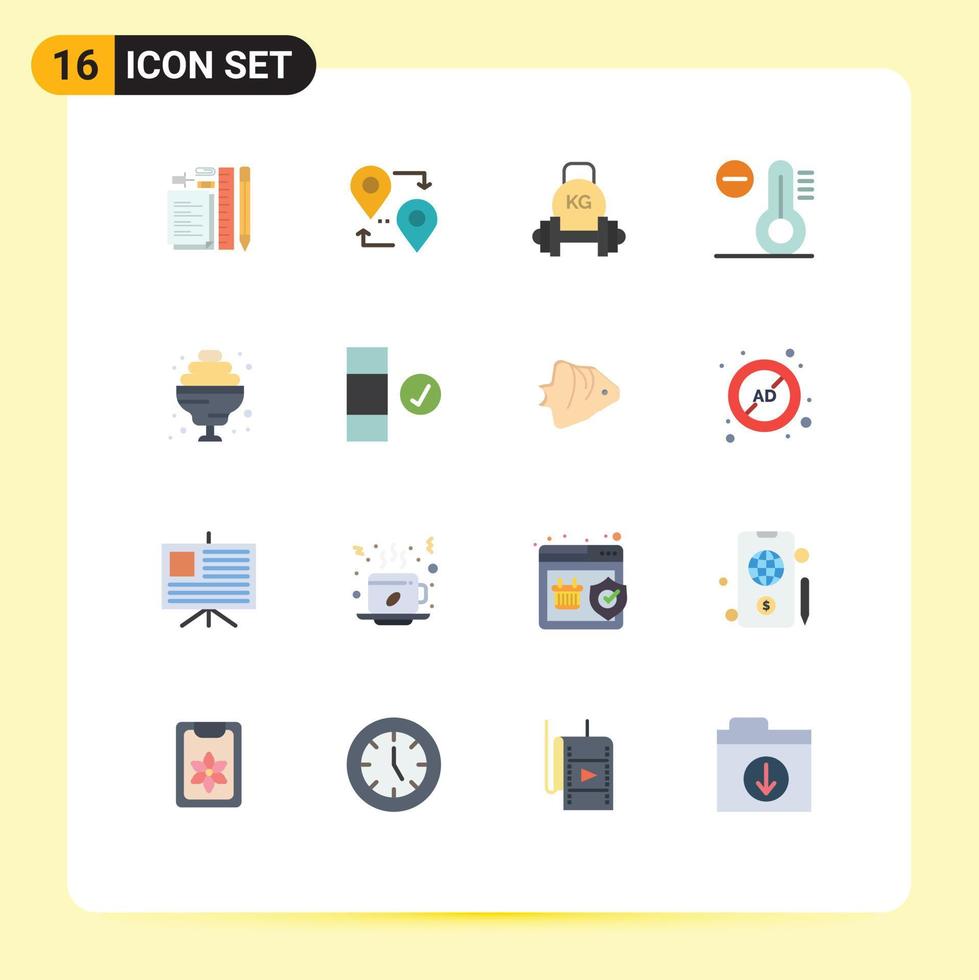The image is a poster featuring 16 stylized, computer-generated icons, each uniquely designed and colorful, evenly spaced out on a white background with a light yellow border. At the top left, the text "16 Icon Set" is prominently displayed. The icons are organized into four rows and four columns.

In the first row, the icons include:
1. Office supplies such as a pencil, ruler, and paper.
2. Two pinpoint shapes encircled by arrows.
3. A black barbell with a "kg" sign.
4. A stylized thermometer with a minus sign.

The second row contains:
1. A footed dish with a beige or yellow content.
2. A rectangle with three blue stripes and a green checkmark.
3. A fish.
4. A red circle with the word "ADD" crossed out.

The third row features:
1. A flag on an easel.
2. A cup of coffee.
3. A shield with a green checkmark on a screen.
4. A rectangular object with a dollar sign and a pen.

The final row includes:
1. A clipboard with a peach-colored paper and a pink flower.
2. A clock showing approximately 5 o'clock.
3. A roll of film with a red arrow.
4. A folder with a download arrow.

These icons are designed to be visually instructive and could be suitable for use in educational or creative office environments.